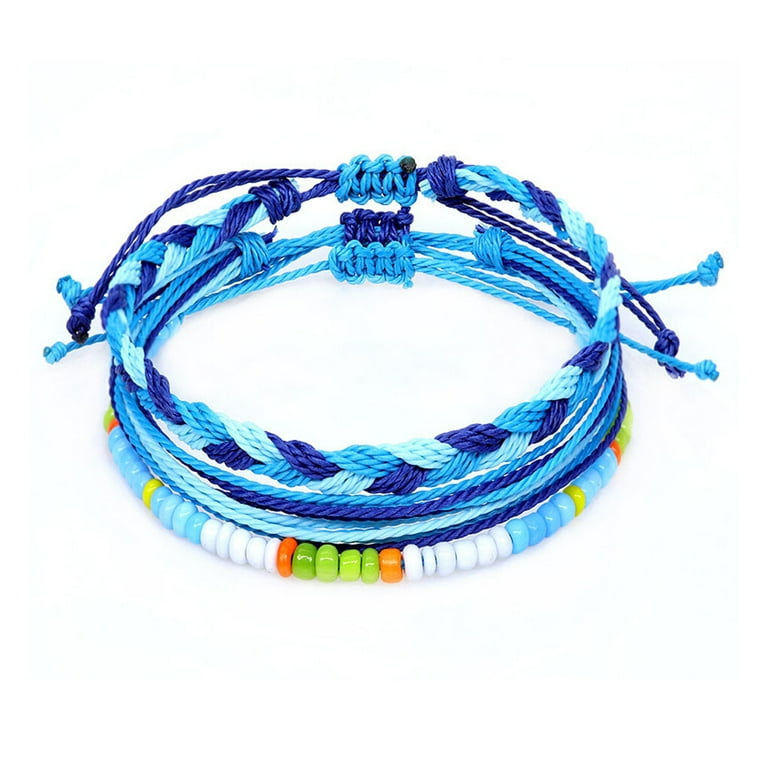This photograph features an array of handmade bracelets displayed on a white background. The bottom bracelet is predominantly beaded and strung on a blue nylon rope. The beads form a detailed pattern with varying colors, primarily blue, accompanied by white, green, red, orange, and yellow beads interspersed in a specific sequence. Above this, there are several woven bracelets made from yarn, showcasing different shades of blue and turquoise. These woven bracelets are intricately braided, creating a thicker, rope-like strand that gives a cohesive look. The overall display suggests a collection of friendship bracelets, reminiscent of those crafted at camp, with both the beaded and woven elements sharing a harmonious blue-toned color scheme that flows through the entire set.